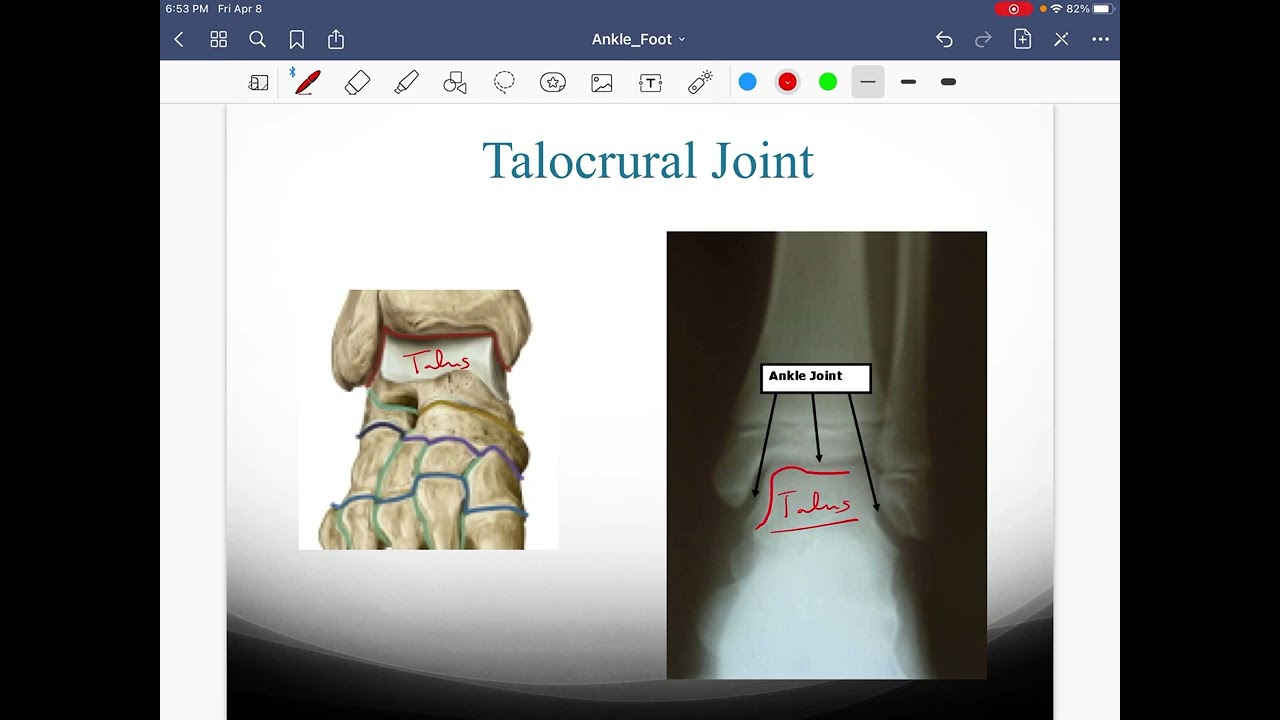The screenshot showcases an image editing software running on a screen, likely a tablet or a phone. At the very top, a horizontal blue strip displays system information: on the left, the time "6:53 p.m." and the date "Friday, April 8," and on the right, the battery percentage "82%", a Wi-Fi indicator, and various status icons. Below this, a dark gray horizontal bar features multiple icons for image editing, including undo, redo, new document, close, and file options like search, bookmark, and share with the title "Ankle_Foot" centered in the middle.

Directly underneath, a white toolbar hosts additional image editing tools. The main section of the screen displays a medical slide titled "Talocrural Joint" in dark green text. The slide comprises two images: on the left, an anatomical illustration of the talocrural joint area with red text labeled "Talos," and on the right, an X-ray highlighting the ankle joint with the same handwritten "Talos" note. The entire image is bordered by vertical black strips on both sides.